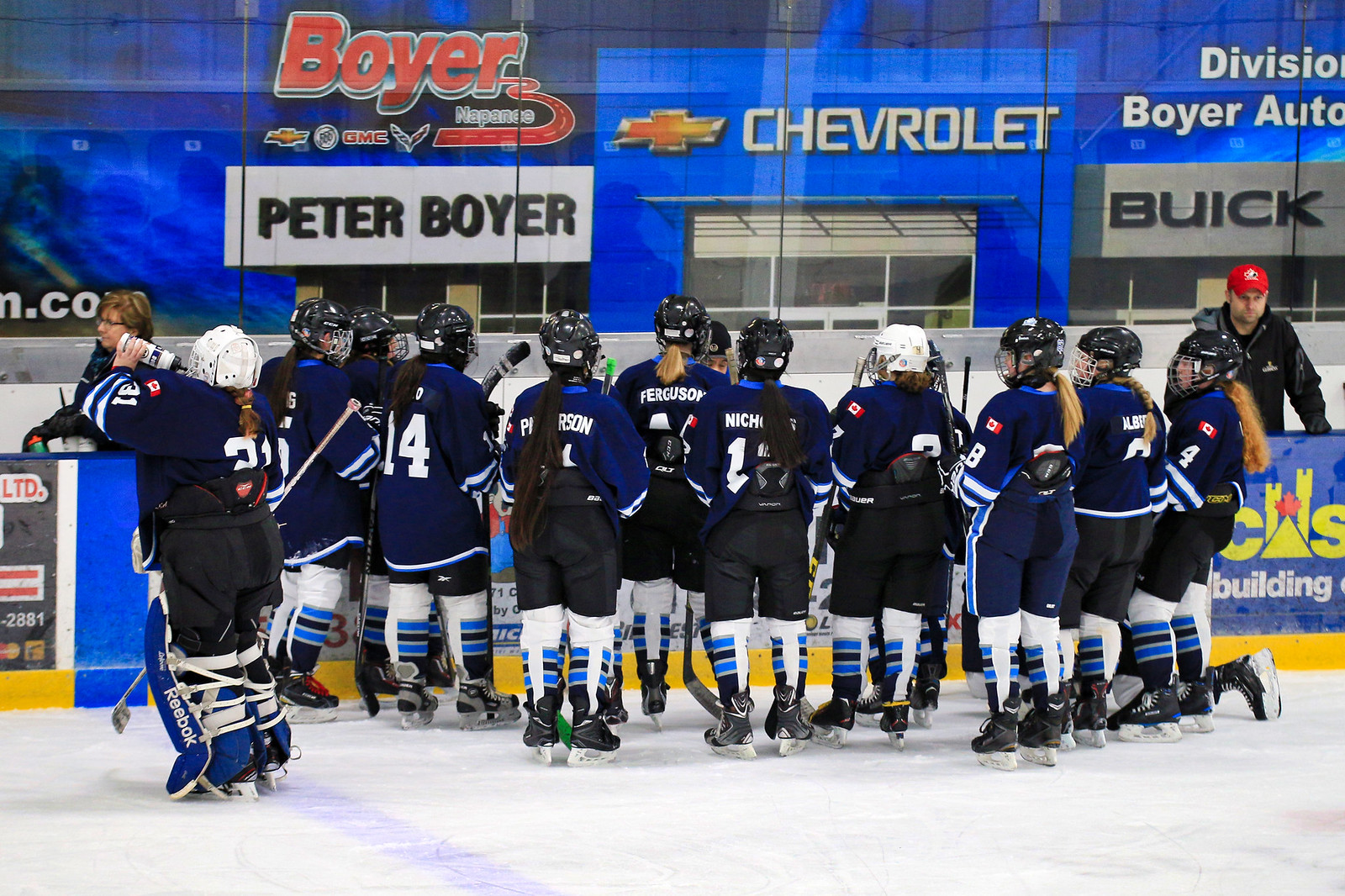In the image, we see a clearly laid-out ice hockey rink, likely located in a sports arena, given the presence of painted lines on the ice. The scene is dominated by a group of female hockey players, approximately a dozen, all huddling near the wall. They are fully geared up in blue and white jerseys, with most of them wearing black helmets, while a couple don white helmets. The players are positioned centrally in the photograph with their backs turned to the camera, engaged in what appears to be a discussion or receiving instructions from someone on the other side of the wall. The rink’s atmosphere is captured with a predominantly blue and white color scheme. Above the players, a series of banners displaying advertisements are visible, including brands like Boyer, GMC, Peter Boyer, Chevrolet, Buick, and CIS Building LTD. Additional details like "Divizio," although partially obscured, contribute to the scene's overall commercial feel. The setting is indoors, suggesting it is either during a game or a practice session.